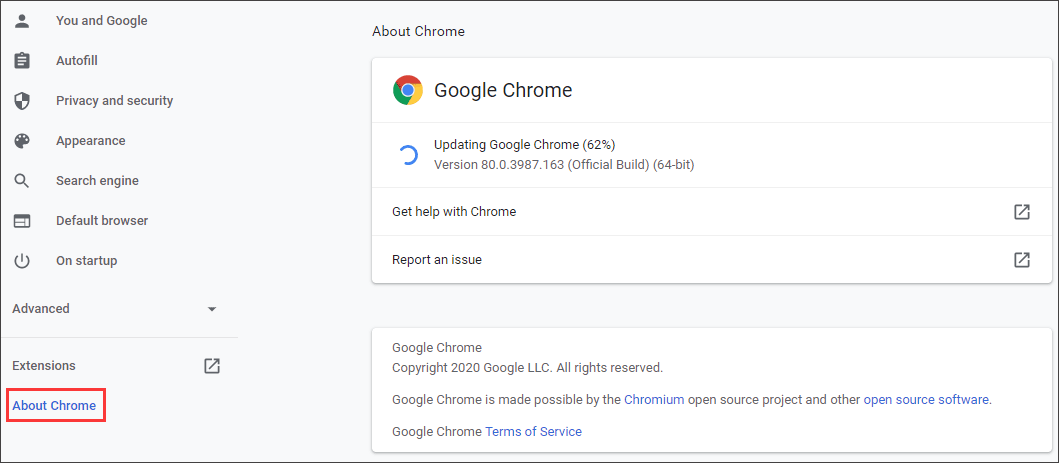The image showcases a Google Chrome settings page in the midst of an update, with the progress bar indicating that the update is at 62%. On the left-hand side, a navigation menu lists various settings categories: "You and Google," "Autofill," "Privacy and Security," "Appearance," "Search Engine," "Default Browser," "On Startup," "Advanced," and "Extensions." The "About Chrome" section is highlighted with a red rectangle. At the bottom of the page, there's a note that reads, "Google Chrome is made possible by the Chromium open-source project and other open-source software," underscoring the collaborative and freely distributed nature of the software. The user appears to be examining Chrome's settings, although their exact intentions remain unspecified.